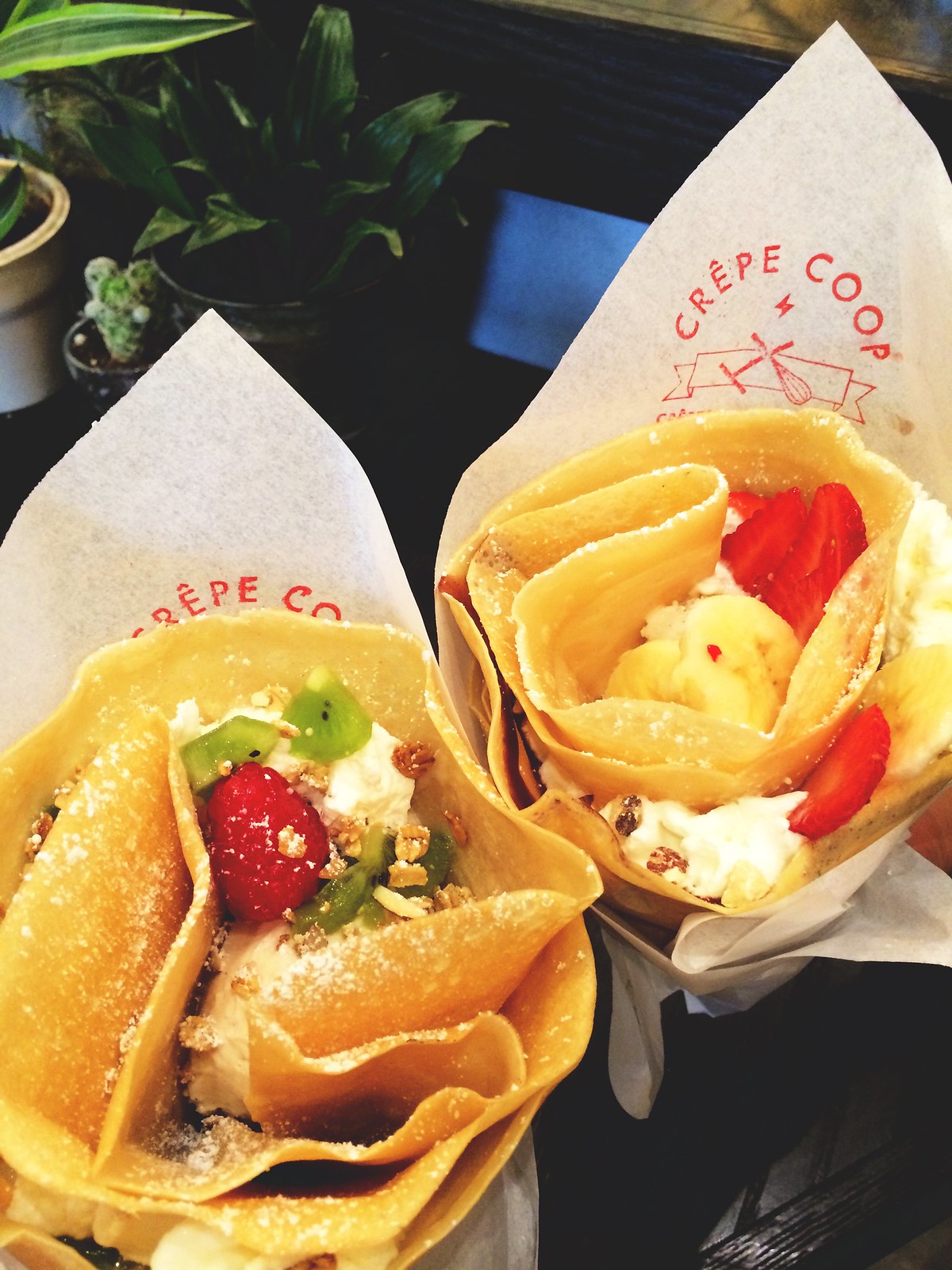This is a close-up photograph of two sweet crepes from a company called Crepe Co-op, displayed upright and wrapped in white paper adorned with "Crepe Co-op" in red letters. The light brown crepes, resembling cones, have a thin pastry layer filled with layers of cream, fruit pieces, and nuts. The crepe on the left contains ricotta, raspberry, kiwi, and crushed nuts, while the one on the right is filled with banana, strawberry, cream, and nuts. Both crepes are dusted with powdered sugar. In the background, three green plants are visible against a dark backdrop, highlighting the focus on the delectable crepes.